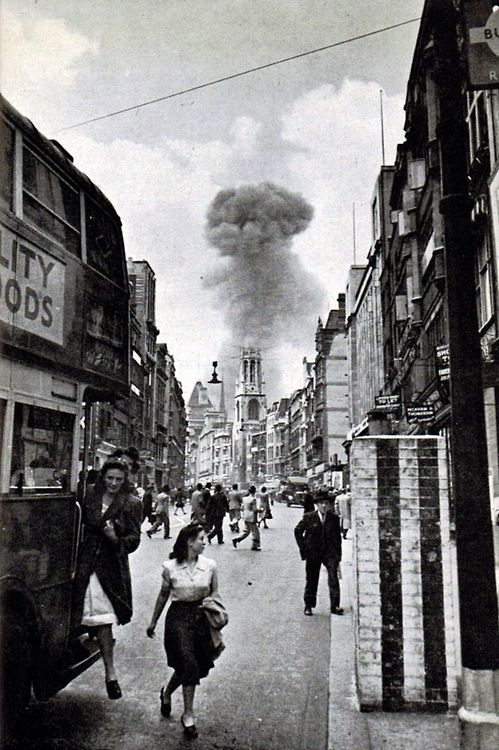This black and white photograph, possibly from the 1930s to 1950s, captures a bustling street scene that appears to be in London, evidenced by the presence of a double-decker bus with the words "City Foods" visible on its side. The scene is filled with numerous pedestrians, including two women getting off the bus. One woman is wearing a jacket, while the other, positioned in front of her, is dressed in a white shirt and skirt. The street is flanked by buildings on both the left and right sides.

Amidst the street activity, an alarming detail emerges in the background: a large plume of smoke billows into the sky, suggesting a fire or an explosion, possibly linked to World War II given the era's historical context. Despite this ominous scene, the people in the foreground appear remarkably unaffected, with nobody turning to look at the smoke or displaying signs of distress. The photograph also captures a power line stretching diagonally across the top right corner against a backdrop of many clouds, adding further to the atmospheric tension of the image.